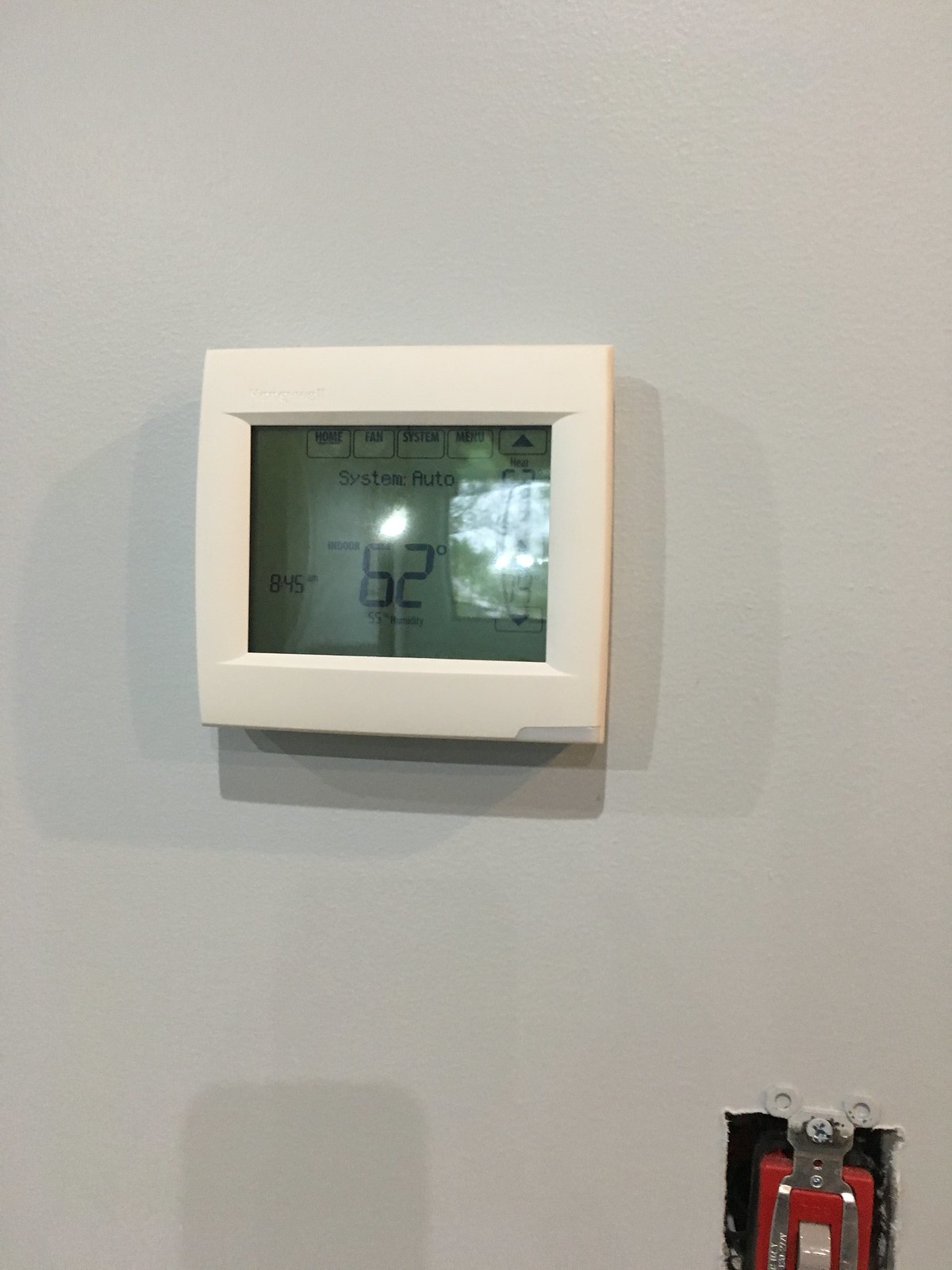This color photograph captures a central wall-mounted thermostat in a clean, well-lit setting. The wall is painted a light gray hue that serves as a neutral backdrop for the main subjects. Dominating the center of the image, the thermostat with its white or off-white plastic casing frames a digital display screen, which prominently shows a temperature of 62 degrees. Above the temperature reading, a series of digital icons and text add informative details. 

To the bottom right of the thermostat, there's an open light switch lacking its plate, revealing the internal metallic components and a red section around the switch mechanism. The white switch itself is partially visible, with its lower portion cut off by the edge of the image. Securing the plate to the wall, a screw is visible, adding to the unfinished appearance of the switch.

Shadows cast by the thermostat create intriguing shapes around it, with additional shadows present at the lower left corner of the image. Reflecting elements of the surrounding environment, the screen of the thermostat displays the faint outlines of a door, a bright window, and trees, adding a subtle complexity. Bright highlights are particularly noticeable around the center-right of the display, just above the 62-degree reading, suggesting a strong light source beyond the window.